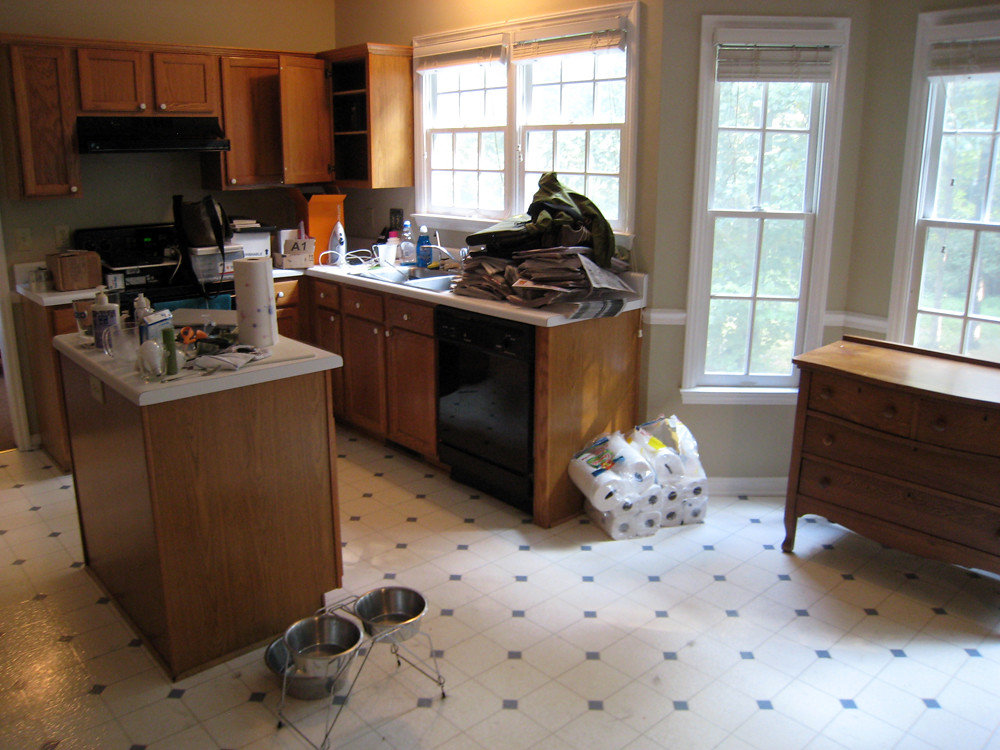In the image, we see a spacious and well-lit kitchen with a detailed and organized layout. The floor is paved with elegant white tiles featuring delicate blue diamond accents at the corners, adding a subtle yet charming touch to the room. The walls are painted a light beige, trimmed with crisp white borders that match the pristine white windows and doorways encircling the space.
 
Prominently positioned is a large, brown wooden dresser brimming with drawers, contributing to the room's storage capability. On the floor nearby, a partially opened large package of paper towels lies open, with a few rolls scattered around. The long, expansive countertop, gleaming in white, offers ample working space and houses a dishwasher with a sleek black front. The brown cabinets beneath provide ample storage and complement the white countertop tastefully.

In the center of the kitchen stands a small island, composed of the same brown wood and topped with matching white, enhancing the kitchen's functionality and aesthetic appeal. The far wall is a hub of activity, adorned with numerous cabinets that offer generous storage options, and a stove integrated into this ensemble.

On the countertops, paper towels, various boxes, and bottles are visible, hinting at a busy kitchen environment. An iron is set up, along with dishwashing liquid in the sink, suggesting multitasking between chores. Additionally, there is a clutter of clothes, magazines, and newspapers piled up on one side, adding a lived-in feel to the room.

Finally, dog bowls are neatly placed on the floor, indicating a pet-friendly household. The overall scene exudes a blend of organization and everyday hustle, making it a warm and welcoming heart of the home.